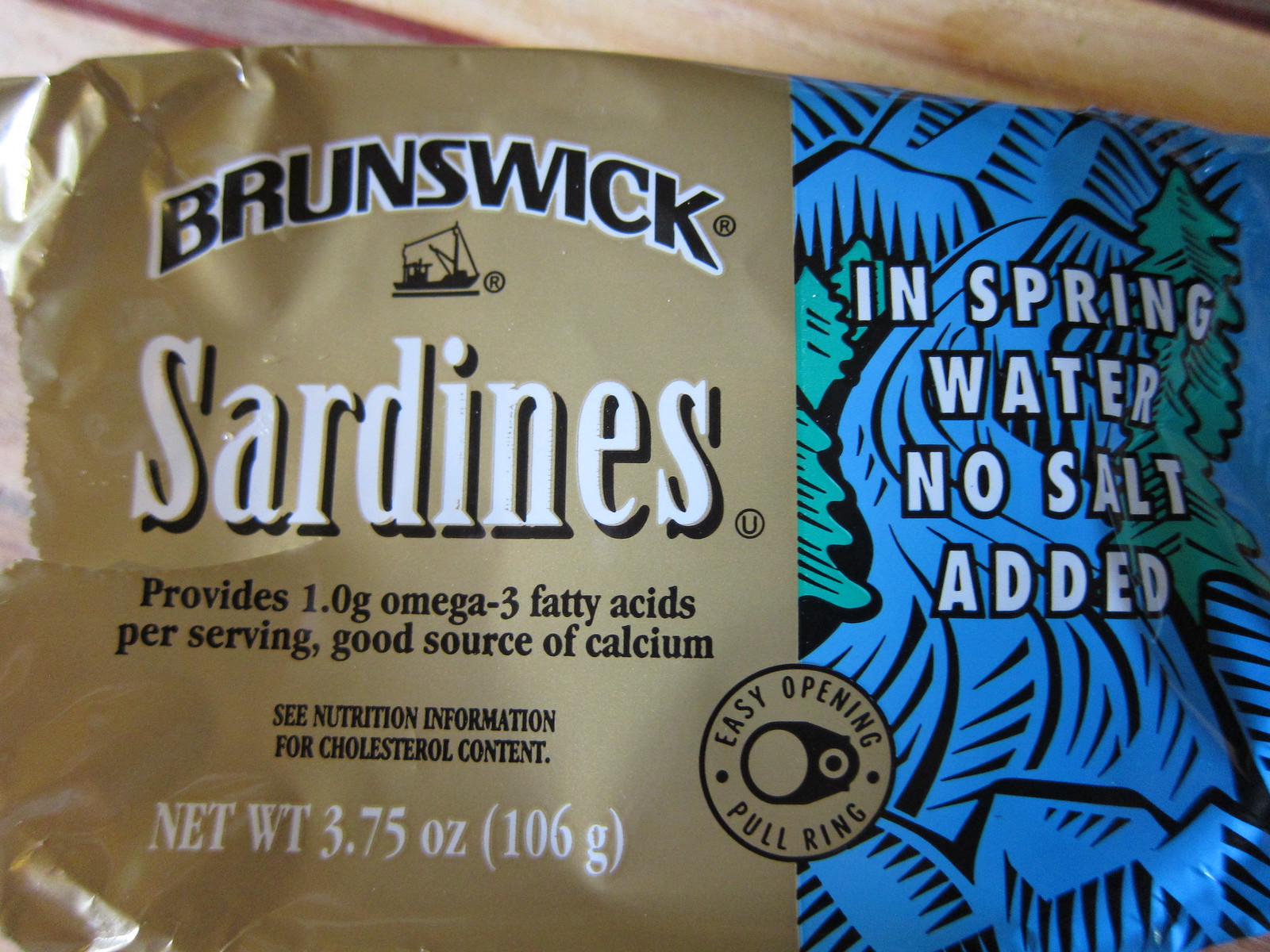This is a close-up photograph of a sardine container, with the packaging divided into two distinct halves. The left side of the package is gold with black and white text that reads "Brunswick" at the top, followed by a silhouette of a fishing boat. Below that, it states "sardines," "provides 1.0 grams of omega-3 fatty acids per serving," "good source of calcium," and mentions to "see nutrition information for cholesterol content." The net weight of the package is 3.75 ounces (106 grams). Within the gold and blue sections, there's a circular icon illustrating an "easy opening pull ring." The right side features an artistic representation of a blue river with mountains and green trees, along with white block letters outlined in black that read "in spring water, no salt added." The package is placed against what appears to be a wooden table background.